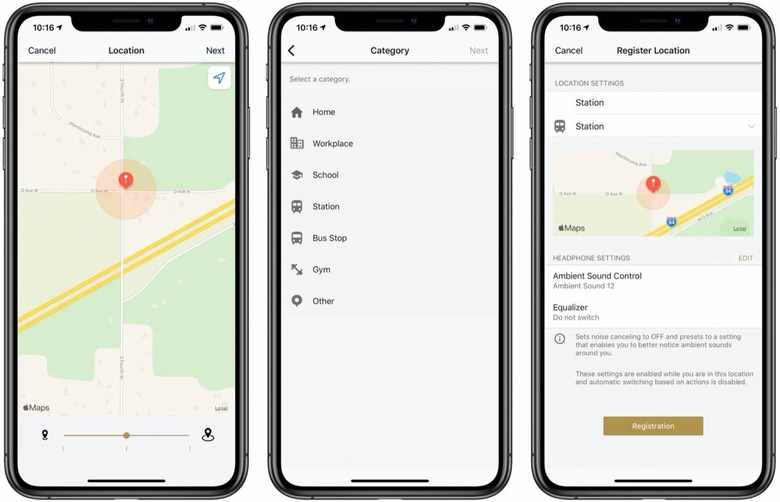This image showcases three smartphones, each displaying a different section of the Google Maps interface with a timestamp of 10:16, featuring send icons, battery indicators, and Wi-Fi icons.

The first smartphone screen shows tabs labeled "Cancel," "Location," and "Next" at the top. Beneath these tabs, you'll find a map with a "You are here" icon, accompanied by a gauge that can be slid left and right.

The screen on the middle smartphone displays a category selection interface. At the top, there's a left-facing arrow for navigating back, followed by category options such as Home, Workplace, School, Station, Bus Stop, Gym, and Other.

The third smartphone screen has a "Cancel" button at the top left and a "Register Location" button below it. It contains sections for "Location Settings," "Station," and a drop-down menu. The map beneath these options also shows a "You are here" icon. Additional settings include Headphone Settings, Ambient Sound Control at level 12, Equalizer, and a "Do Not Switch" option. There is also some small, unreadable text and a final "Registration" button at the bottom.

All three screens feature a home button at the bottom of their displays.